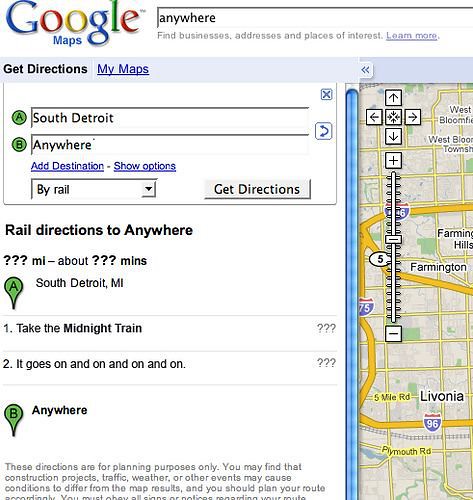Caption:
This image depicts a humorous Google Maps search. The search box displays "anywhere," with "A" marked as "South Detroit" and "B" as "anywhere." Below, there's an option to search for rail directions with placeholders such as "??? miles" and "??? minutes" to the destination. The text whimsically references the song "Don't Stop Believin'" by Journey, mentioning "Take the midnight train" and the lyrics "It goes on and on and on." Additionally, there's a small inset map on the right showing streets and nearby locations like Farmington and Livonia, but without any specific directions or markers. This image is a playful nod to the iconic song lyrics and the idea of traveling to an undefined destination.